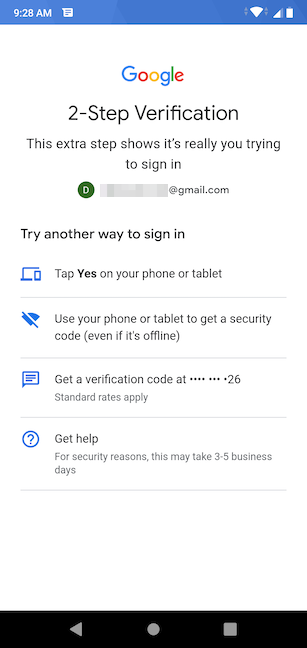Screenshot of a cell phone displaying a two-step verification prompt. The top blue bar indicates it's 9:28 AM, and it shows full Wi-Fi signal, nearly full carrier signal, and a nearly depleted battery. On the right side of the bar, there are gray icons for an up arrow, a down arrow, and an up-and-down arrow.

The main content area begins with the Google logo in its classic colors, followed by a notification for two-step verification, which states: "This extra step shows it's really you trying to sign in." Below this, there's a black circle with a 'D' in it, representing a user profile.

The user's email address is partially redacted: "name@gmail.com." Under this, options for alternative sign-in methods are presented, starting with a message suggesting to "Try another way to sign in." There are icons for a blue computer and a blue phone, indicating that you can "Tap yes on your phone or tablet."

Following a gray line separator, there's a blue Wi-Fi icon with a line through it, alongside instructions to use your phone or tablet to get a security code even if offline. Another gray line separates this section from the next, which mentions receiving a verification code via text message to a partially obscured number ending in "26."

The phrase "Standard rates apply" follows, after another gray line. Next, there is a blue circle with a blue question mark inside it next to a white circle with the text "Get help." A note at the bottom informs users that for security reasons, this process may take three to five business days.

Finally, at the bottom of the phone screen, there's a black navigation bar with gray icons for a triangle, a circle, and a square.